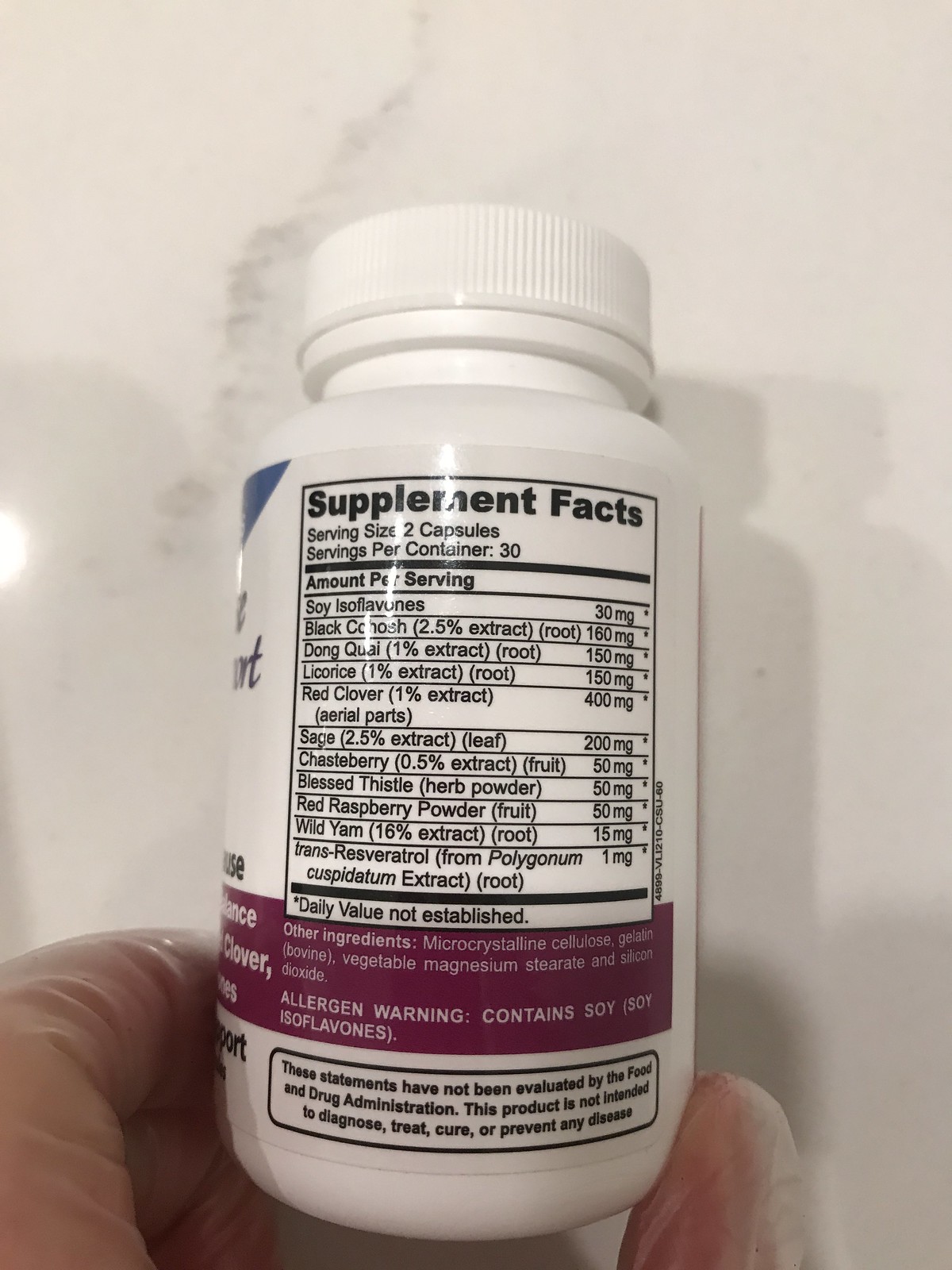A white bottle of herbal supplement tablets is being held by a person wearing a latex glove against a light gray wall with a darker streak. The bottle, circular with a white lid, features a label providing supplement facts in black print over a white background. A prominent purple banner runs across the middle, with additional details at the bottom in black. The label specifies a serving size of two capsules, with 30 servings per container. Key ingredients listed include soy at 30mg, red clover extract at 400mg, wild yam at 15mg, black cohosh extract at 160mg, dong quai root extract at 150mg, and licorice root extract also at 150mg.